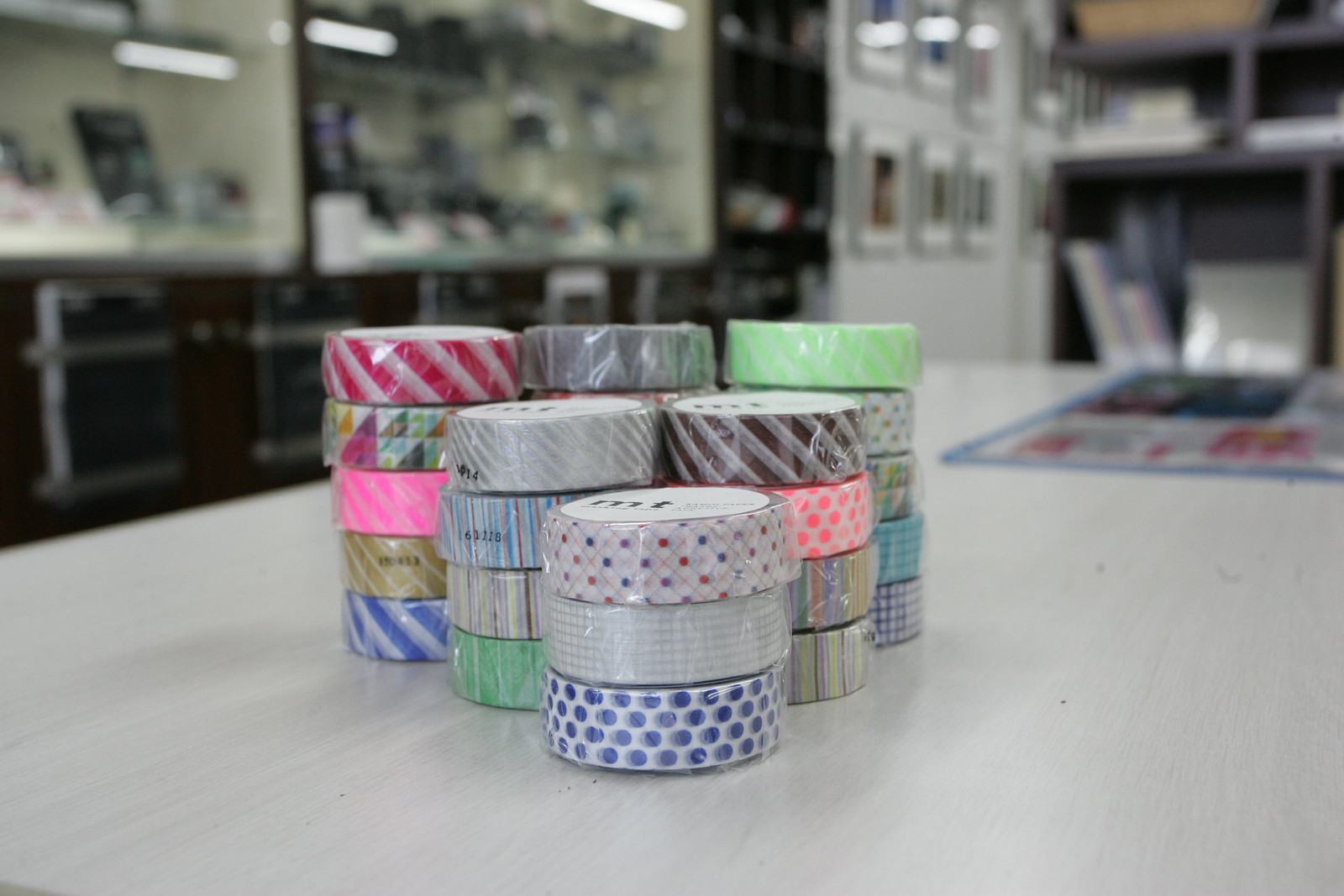This image captures a detailed close-up of a craft store display, focusing predominantly on an assortment of colorful washi tapes and ribbons meticulously stacked on a light gray countertop. In the foreground, three main piles of ribbons form a triangular arrangement: the closest pile consists of three layers of ribbons with distinct designs, including polka dots and checkered patterns in hues of blue, gray, and red. Just behind it, there are two columns, each with four stacked ribbons of various colors and patterns like silver stripes, blue and purple stripes, and polka-dotted designs in shades of pink and green. Farther back, three columns of five ribbons each feature an array of vibrant designs, including stripes, polka dots, and checks in colors like bright pink, lavender, golden, and blue stripes.

The background reveals a blurry scene with a white wall adorned with two rows of artwork and a gray shelf immediately behind the countertop. Several black cabinets with white shelves, containing lined-up objects like books and notebooks, add to the organized yet creative ambiance of the store. The entire setting is brought together with a subtle blend of gray and white tones, enhancing the vibrant display of crafting materials at the forefront.